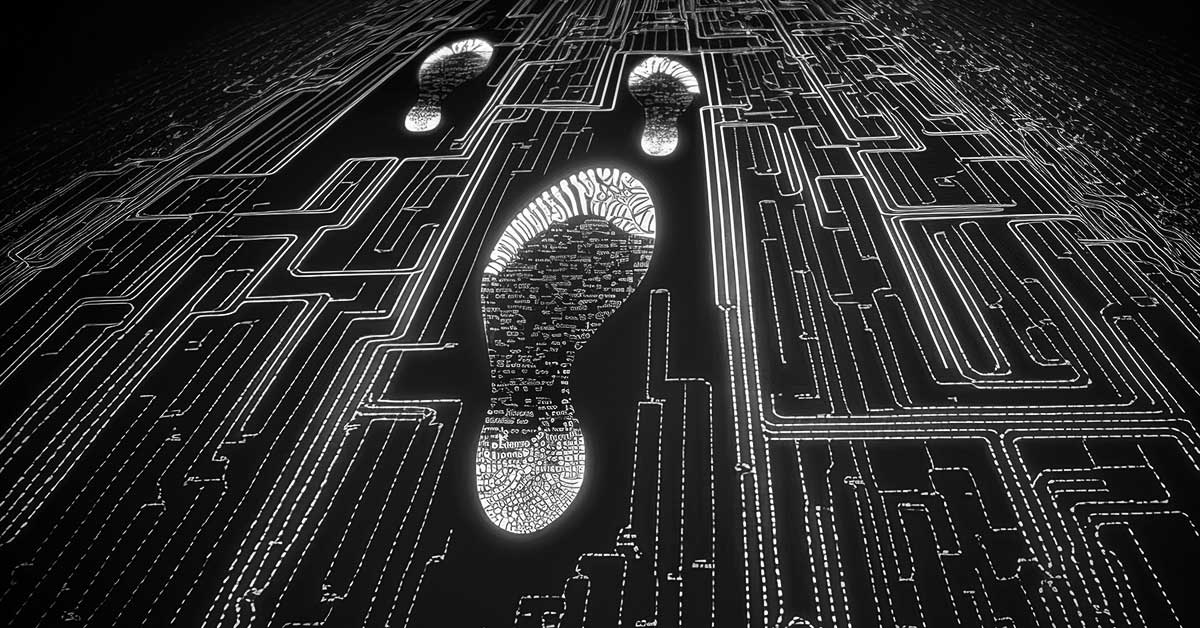This black and white digital illustration depicts a high-contrast black background illuminated by white geometric lines resembling a printed circuit board or motherboard. In the foreground and narrowing towards the background, these intricate white lines and dotted wires create a perspective effect, emphasizing the depth of the image. Central to the composition are three detailed shoe prints, arranged in a specific layout: one prominent footprint in the center, another above it, and a third smaller print to the top left. The footprints themselves are striking, composed of technical lines and irregular white shapes for the toes and heel, conveying a sense of digital or computerized footprints. The image exudes an aura of security and technology, enhanced by the stark black corners and the intricate pattern of white lines resembling lines of code.